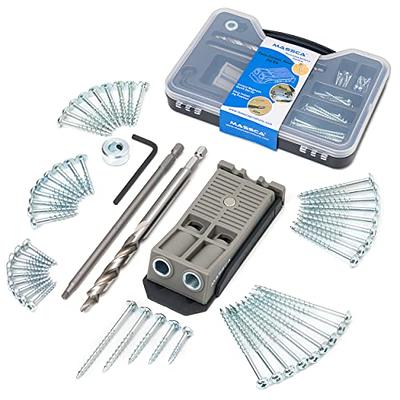This photograph depicts a well-organized toolkit featuring a variety of tools and fasteners essential for DIY or professional use. At the center is a plastic case with a clear lid, allowing visibility of its contents. The case is black with a blue and white cardboard label wrapped around it, which is slightly unreadable but contributes to its branded look. Inside the compartments of the case are neatly arranged screws, nails, and different sizes of drill bits. Additionally, the toolkit includes Allen wrenches and a gray device with silver trim, all arranged in a visually appealing semicircle display beneath the case, making it ideal for advertisement purposes. The whole setup showcases the comprehensive tool assortment and highlights the precise organization and variety of items included within this versatile kit.